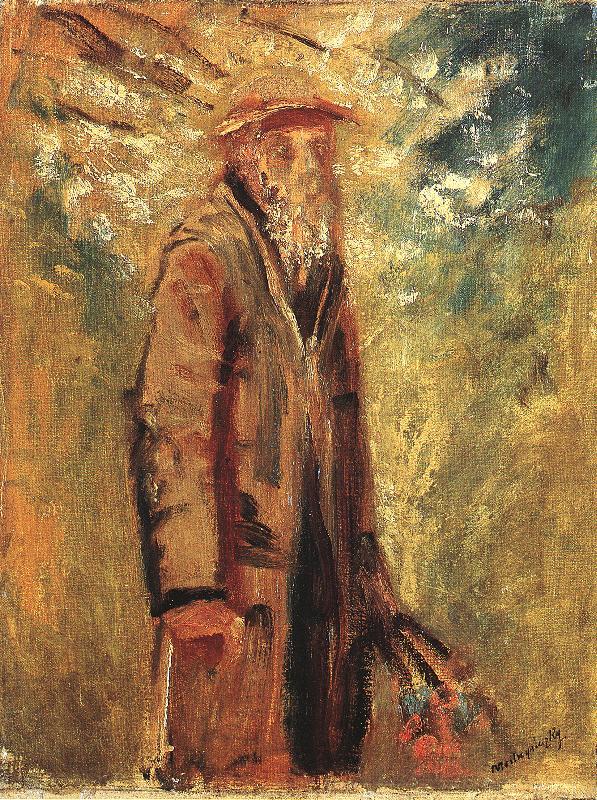The painting features a roughly rendered portrait of an elderly gentleman standing in profile, enveloped in warm, dark overtones. The background is a blend of orange-brown hues, transitioning to darker shades of green and blue in the upper right-hand corner. The man's figure is prominently captured with rough brushstrokes, giving it a somewhat abstract quality. He wears a long brown overcoat outlined in black, open to reveal similarly colored garments beneath. His hat, also brown, and his mottled gray beard enhance his aged appearance. In his left hand, he holds an indistinguishable item—possibly a bouquet of roses or a case—angled downwards. Despite the unclear details of his face, there is a solemn aura about him, almost suggesting a sense of melancholy. The artist's signature is located in the bottom right corner, rendered in black, yet it remains undecipherable. The overall composition, with its amalgamation of mottled golds, browns, grays, and hints of green, evokes a contemplative atmosphere, making one ponder the man's purpose and story within this evocative scene.